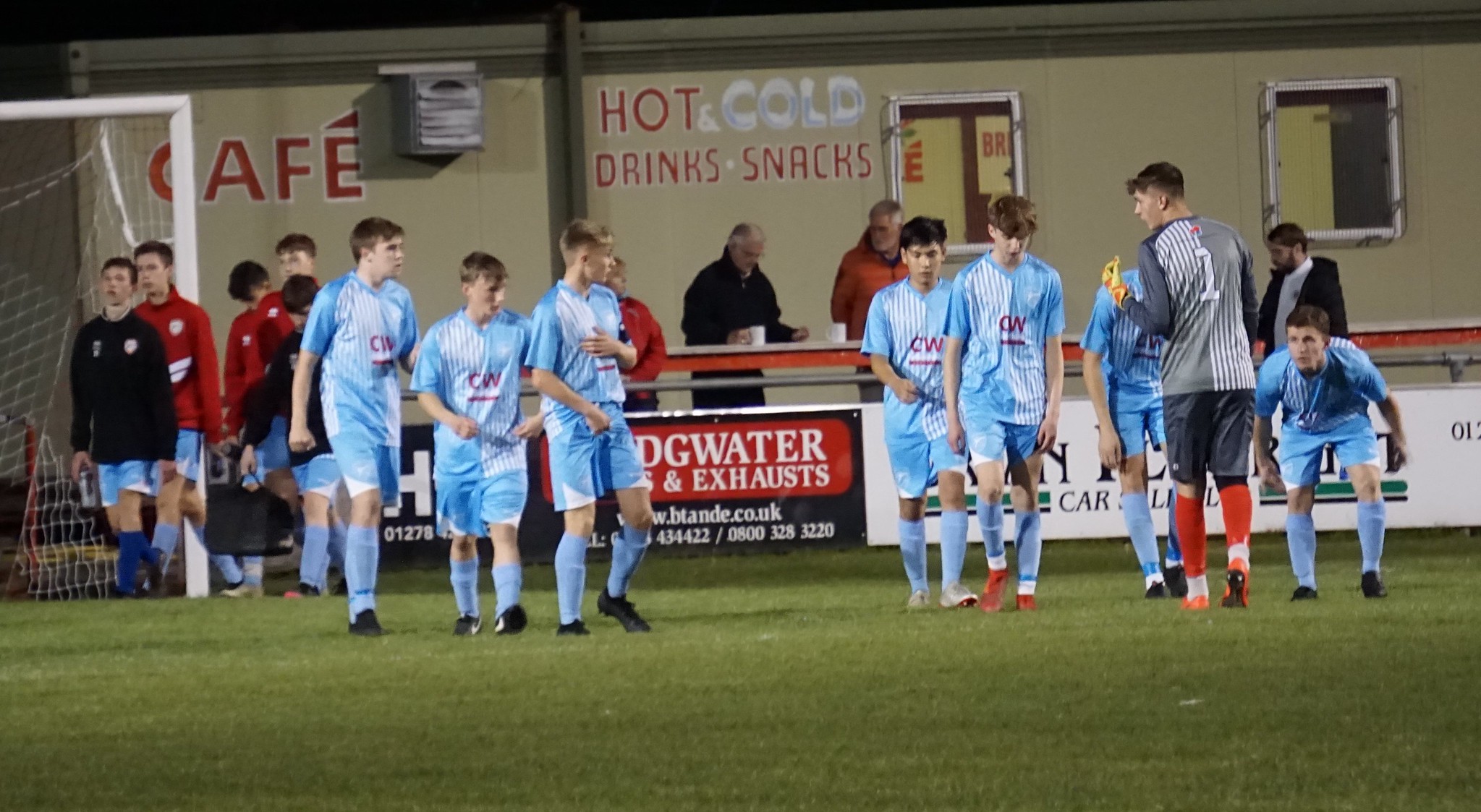The image captures the moment before the start of a boys' soccer match on a grassy field. In the foreground, there is a section of the soccer goalpost visible on the left side, with two young boys standing in front of it—one dressed in black and red, both wearing blue shorts. The main focus is on a group of boys in uniforms, centered on the field. On the left, three boys are dressed in blue shirts, shorts, socks, and black shoes. To the right, four more boys wear similar blue and white shirts, shorts, and blue socks. Facing the players is a young man in a referee's uniform with a black-and-white vertically striped shirt, gray sleeves, gray shorts, and orange socks. In the background, a one-story white building marks the border of the field. The building features signage that reads "café" and "hot and cold drinks and snacks." In front of the building is a long table, with people standing behind it. There is a short wall with advertisements separating the table from the field, and various individuals, possibly coaches, parents, or other players, are walking around, creating a bustling pre-game atmosphere.